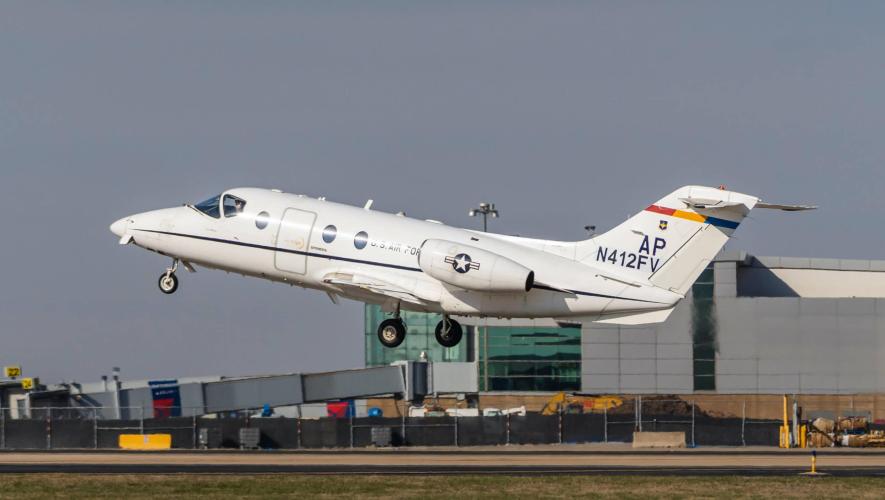This photograph captures a moment when a small, white personal jet, bearing the US Air Force insignia, is in the midst of takeoff from the right side of the frame to the left. The aircraft, possibly seating between five to ten passengers, features the tail number "AP N412FV" and a small strip of red, yellow, and blue colors on its tail. The plane is positioned centrally, with its landing gear visible and three passenger windows seen on the fuselage. In the background, there is a large terminal building with glass panels, hinting at an airport or possibly an Air Force base. A walkway, associated with Delta, and some colorful posters are also discernable. In front of the terminal stands a fence, hinting at the airport's perimeter, with a black strip of runway partially visible. The very foreground of the image is grassy, adding a touch of green to the scene.